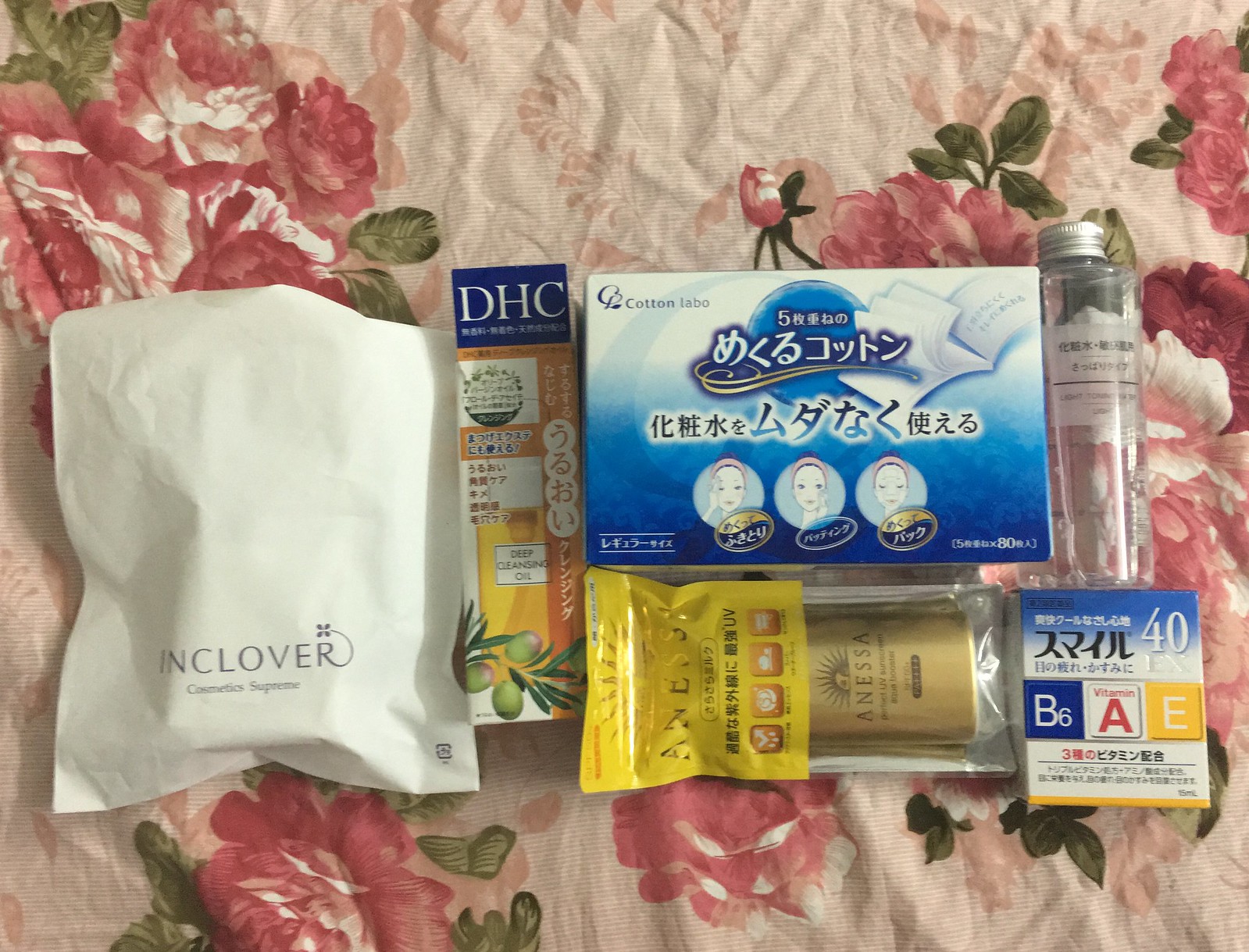This is a color photograph featuring an assortment of cosmetic and personal care items arranged on a slightly crumpled beige floral cloth. The cloth itself is adorned with large, reddish-pink and white flowers accompanied by green leaves, and has an embossed design that adds texture and depth.

On the left side of the image, there is a white pouch, which appears to contain a rectangular object not visible from the outside. The pouch is labeled with black text that reads "in clover," followed by smaller, unreadable text. Adjacent to the pouch is what looks like a cardboard box with a blue edge at the top, bearing "DHC" in white letters. The rest of the box features a yellow and green design with additional green leaves at the bottom and white panels with some illegible black and green text.

Moving to the right, there is a rectangular packet, possibly tissues, with a blue lower section and a white upper section, topped with a logo in eastern script. At the bottom of this packet are three circular images of women's heads alongside unreadable white text.

Below this packet is a sachet placed horizontally. It has a yellow bottom section with black text, and a transparent top section revealing a gold tube with black text inside. Further right is a square item also featuring eastern writing, with circles displaying "B6A" and "E," hinting that it might be related to vitamins or supplements. Above this square item is a clear tube with a silver cap, labeled with a white sticker containing some unreadable black text.